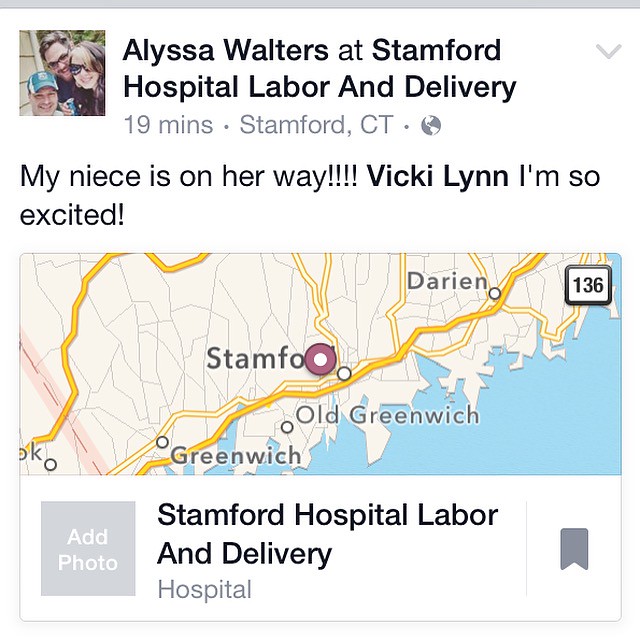This is a color image of a screenshot from a Facebook post by Alyssa Walters, located at Stamford Hospital Labor and Delivery in Stamford, Connecticut, 19 minutes ago. The post enthusiastically announces, "My niece is on her way, Vicky Lynn, I'm so excited," with "Vicky Lynn" tagged in bold, implying she is possibly the mother of the child. Featured in the post is a small photo in the top left corner showing three people, and a prominently displayed map of Stamford, Connecticut with the hospital's location highlighted. The map, which extends from the left to the right of the image, shows Route 136 that connects Stamford with nearby Darien and Old Greenwich. The post is formatted like an ad, with a logo resembling a bookmark in the bottom right corner and another logo in the bottom left, presenting itself as a typical Facebook interface with details about the setting and colorful elements in white, tan, yellow, red, black, and a hint of blue.